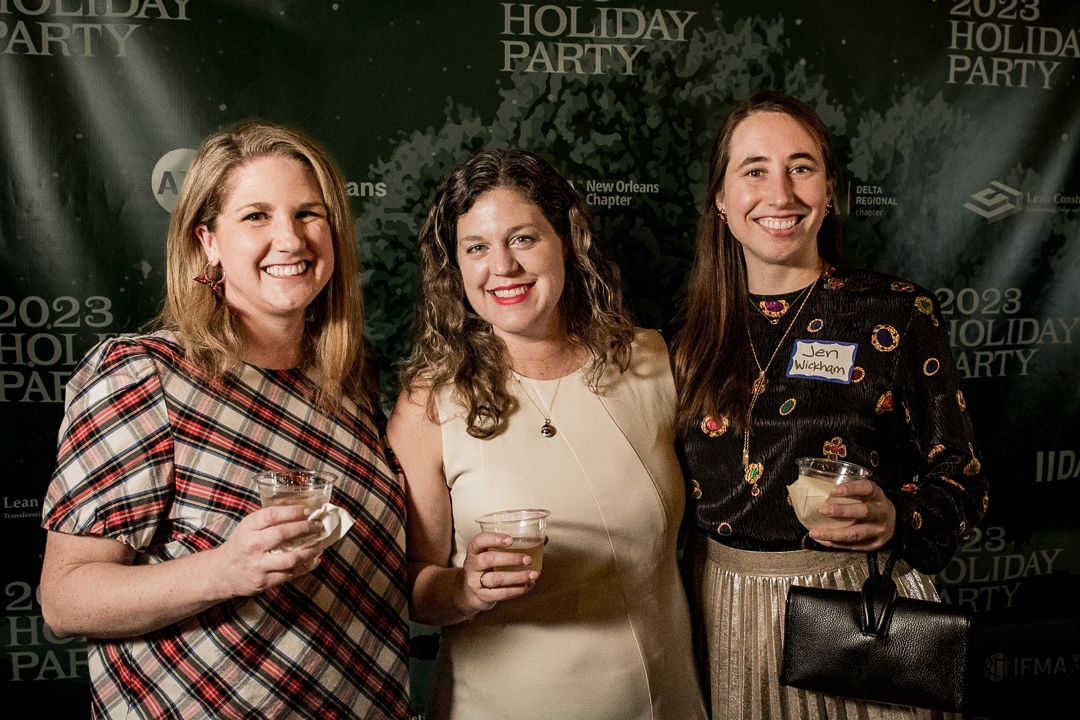The image captures three women standing shoulder to shoulder, smiling and posing with small plastic cups in hand. They are in front of a black backdrop that repeatedly features the text "2023 Holiday Party" in gray, also indicating a connection to the "New Orleans chapter" and "Delta Regional." The woman on the left wears a checkered shirt in black, red, and beige hues, with shoulder-length blonde hair. The woman in the middle dons a tan-colored sleeveless dress, accessorized with a small pendant necklace, and has slightly longer than shoulder-length curly brown hair. On the right, the woman identified by her name tag as Jen Wickham sports a black top with decorative patterns, a shiny tan skirt, and straight chest-length brown hair. They are evidently enjoying the event, captured in a candid moment of festivity and camaraderie.